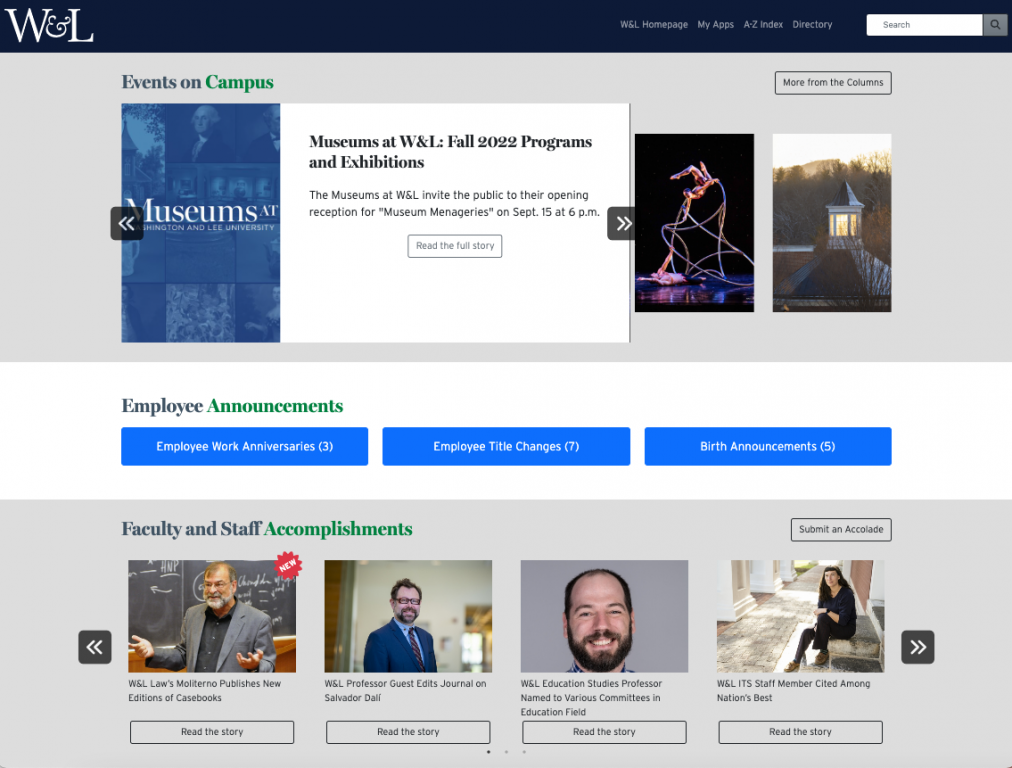The webpage header features a dark blue banner on the top left corner showcasing "W&L" in bold white letters. Adjacent to this are several navigational tabs labeled "Homepage," "My Apps," "Index" with the number 8, "Directory," and a search box. Below the header, there is a section titled "Events on Campus" set against a gray background, which displays various scrollable items.

Currently highlighted is a notice for "Museums at W&L Fall 2022 Programs and Exhibitions," inviting the public to an opening reception for "Museum Menageries" on September 15th at 6 PM. Navigational arrows on each side allow users to browse through different event images.

Beneath this section, there's a segment labeled "Employee Announcements" featuring three blue boxes. These boxes are titled "Employee Work Anniversaries," "Employee Title Changes," and "Birth Announcements."

Further down, the page highlights "Faculty and Staff Accomplishments," displaying four images with articles about these achievements. Above this segment, there is an option to "Submit an Advocate," accompanied by arrows for navigation.